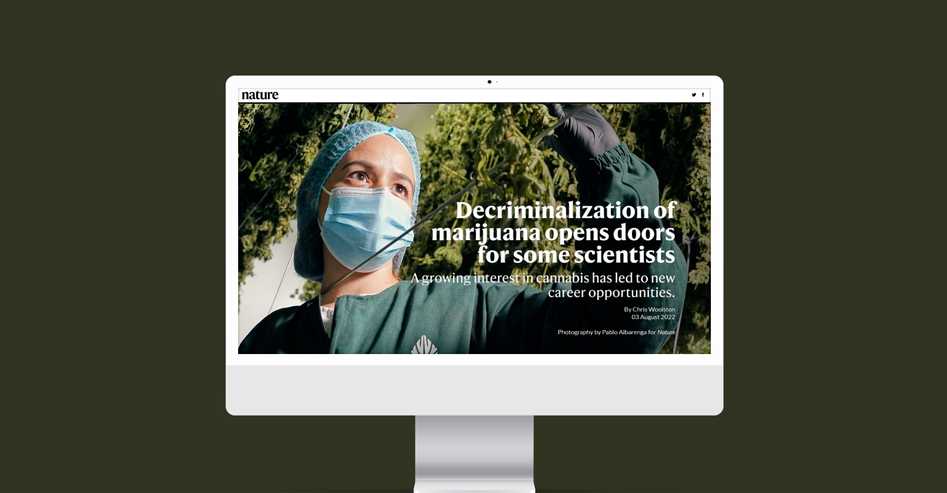The image features a digitally generated representation of an iMac computer set against a black background. The computer screen displays a website titled "Nature" in black font at the top left corner. The main visual focus on the screen is a detailed article about the decriminalization of marijuana. The article is titled "Decriminalization of Marijuana Opens Doors for Some Scientists" and is followed by a subheading that reads, "A growing interest in cannabis has led to new career opportunities."

Prominently displayed within the article is an image of a healthcare worker wearing a cap, mask, long sleeves, and gloves, carefully observing a marijuana plant. The worker's attentive stance highlights the scientific and professional approach to studying cannabis. The article credits Chris Woodson as the author, with the publication date marked as August 3rd, 2022. Although the photograph credit appears on the screen, the exact name of the photographer is unclear due to slightly blurry text.

The iMac itself is depicted in a sleek, silvery-white finish, embodying a minimalist design that accentuates the digital content displayed on the screen. The overall composition of the image draws attention to the intersection of technology, scientific research, and the evolving landscape of cannabis studies.